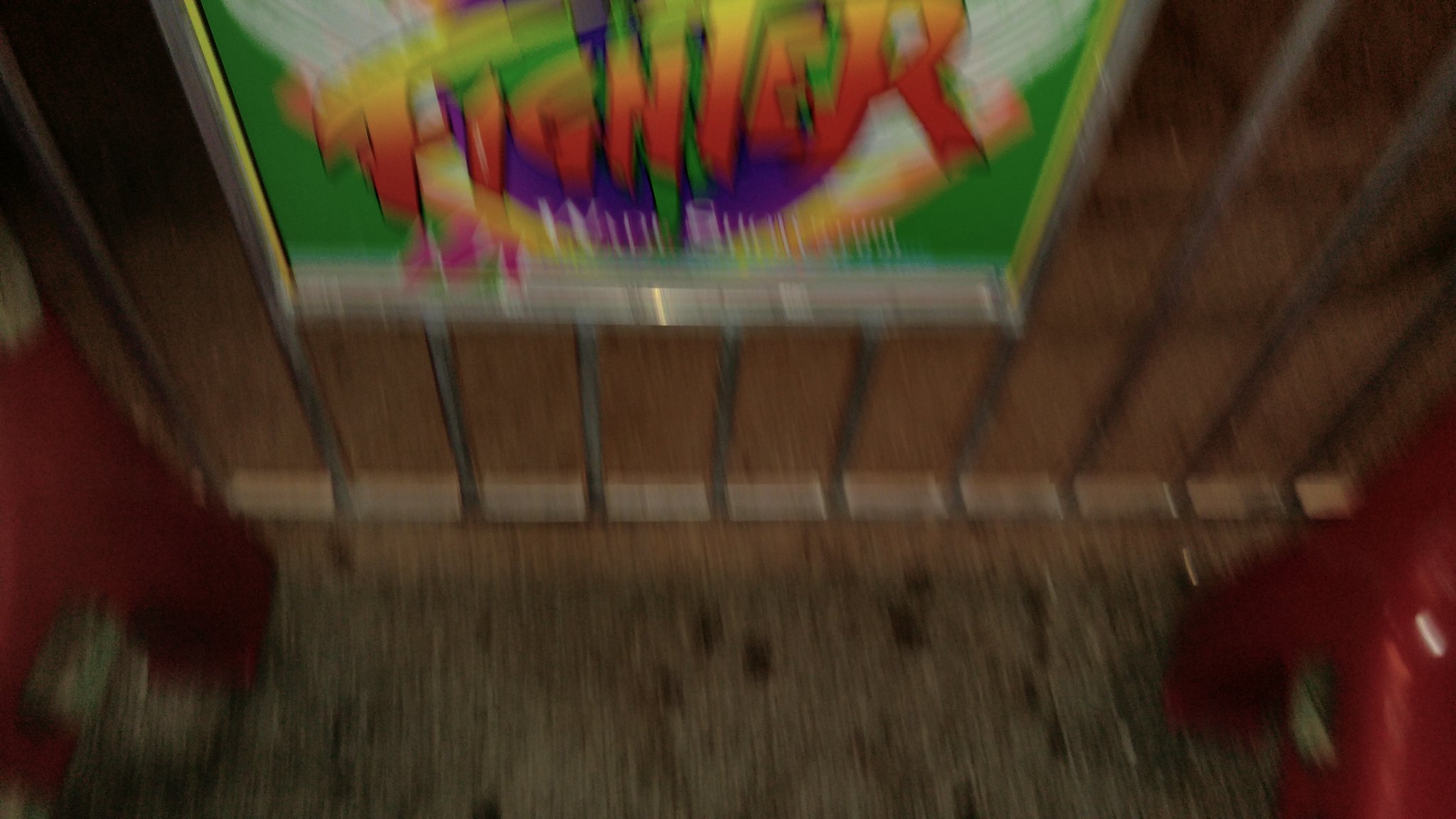This is a color photograph taken at night, characterized by noticeable blurriness that obscures fine details. The shot is angled downward, focusing on the ground below. Prominently in the frame, metallic railings run vertically from the top towards the middle, ending just above the ground where a horizontal line marks their termination. 

Centered slightly to the left on these railings, there is a large, vibrant poster. The poster features a green base gradually transitioning to white at the top. The central section is filled with blurred, multi-colored text in hues of red, yellow, and green, likely spelling out "HIRTIGNIER." Just beneath the lettering is a purple background, decorated with a circular motif, accented with a splash of pink in the lower left corner.

The ground beneath the railings is greyish in tone, illuminated by artificial lighting visible through the bars. Flanking the railings on both the left and right sides, there are indistinct red objects resting on the ground.